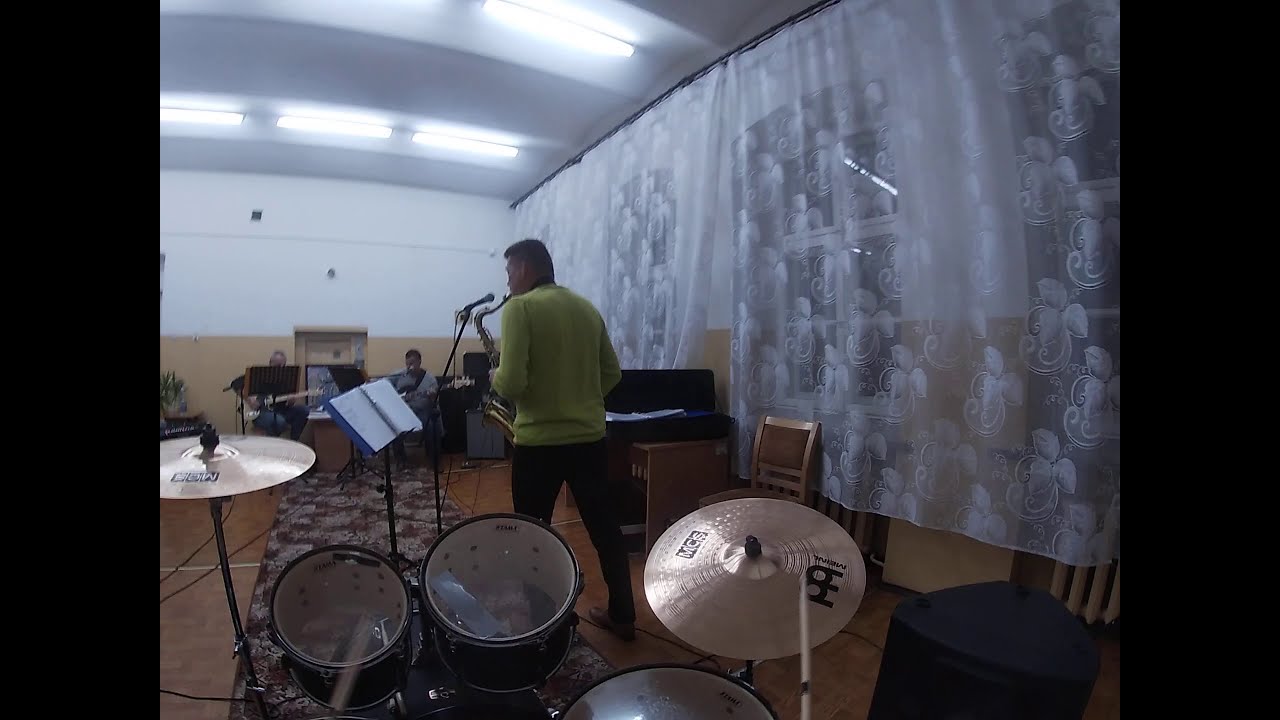In a spacious, well-lit room adorned with large lights crossing the ceiling, a lively practice session or performance unfolds. At the center of the image, a man with short, cropped hair is absorbed in playing an alto saxophone, donning a light greenish-yellow long-sleeve shirt. Positioned near a microphone and looking down at a low music stand, he creates a focal point with his music. Directly in front of him, partially obscured, a drummer is energetically playing, captured from the drummer's vantage point by the presence of two cymbals and blurred drumsticks in motion. To the saxophonist's right, a translucent curtain partially veils large windows, letting in natural light that contrasts with the opaque white walls and a beige lower portion.

Further into the background, more musicians contribute to the ensemble: one, possibly two, individuals can be seen playing guitars or a bass, and another person is near what appears to be a keyboard. Tying the scene together is a small maroon rug with light-colored patterns under the drum kit, laying over the brown wooden floor, enhancing the room's warmth. All participants are engrossed in their respective instruments, creating a dynamic and engaging musical environment.